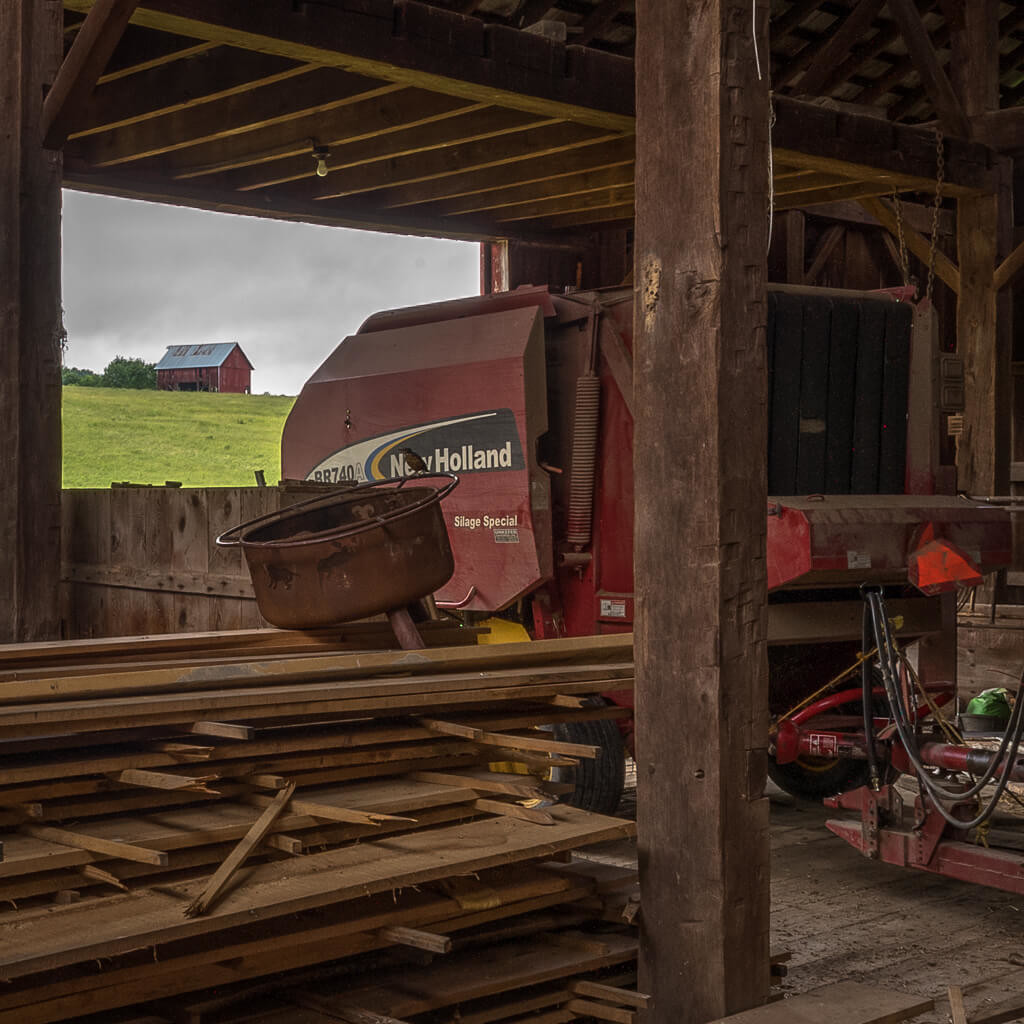The photograph captures a rustic, partially constructed or renovated barn interior, brimming with various textures and warm tones. Dominating the scene is a tall wooden beam standing slightly to the right of center, accompanied by a stack of cut wooden planks and a rusty wash pan or bowl resting on top. The barn floor comprises wooden slats, supported by thick hand-hewn timbers. Adjacent to the beam, a sizable red piece of farm machinery, branded with "New Holland Stage Special," bristles with tubes and hoses, suggesting its function as a harvester or similar equipment.

The back of the barn reveals an open window or doorway, providing a picturesque view of a lush, green hillside topped by another red barn with a metal roof, outlined against a stormy gray sky. This distant barn is slightly elevated, enhancing the sense of depth and rural tranquility in the image. Throughout the scene, the interplay of wooden textures and metal contrasts, depicting a working farm atmosphere poised between timelessness and activity.